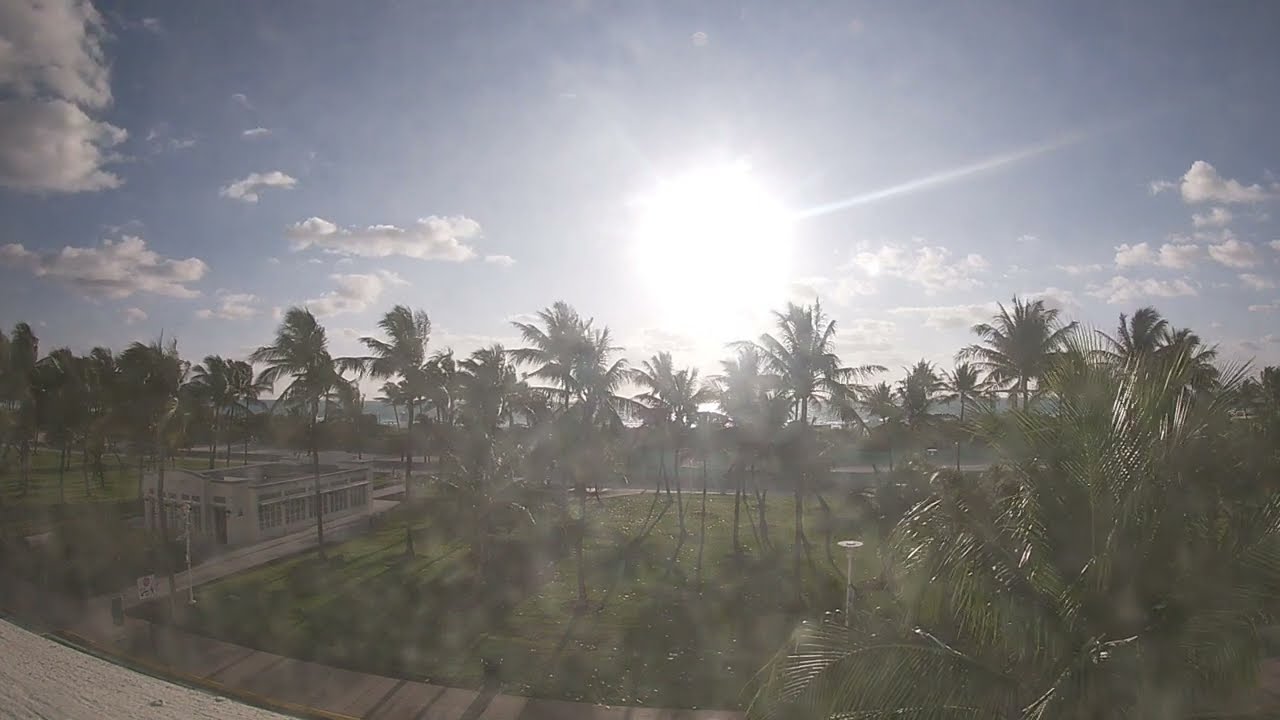This horizontally aligned rectangular image captures an early evening or possibly sunrise scene with a darker blue sky dotted with white and gray puffy clouds. The sun is positioned low in the sky, casting a dramatic light that creates a hazy ambiance. Dominating the lower portion of the image is a large, grassy area populated with numerous palm trees, evoking a tropical setting. A network of sidewalks meanders through this green space, including a main path stretching horizontally across the bottom and a perpendicular walkway intersecting it.

On the left side of the image, partially obscured but visible, stands a white stone rectangular building with an array of square windows. Though slightly blurry, it appears to be a short structure, possibly an office or a small business. In the lower right-hand corner, there's a close-up view of the top leaves of a palm tree. The overall scene suggests an aerial or elevated perspective, perhaps taken from a top floor window, contributing to the bright glare that filters through this serene tableau devoid of people or vehicles.